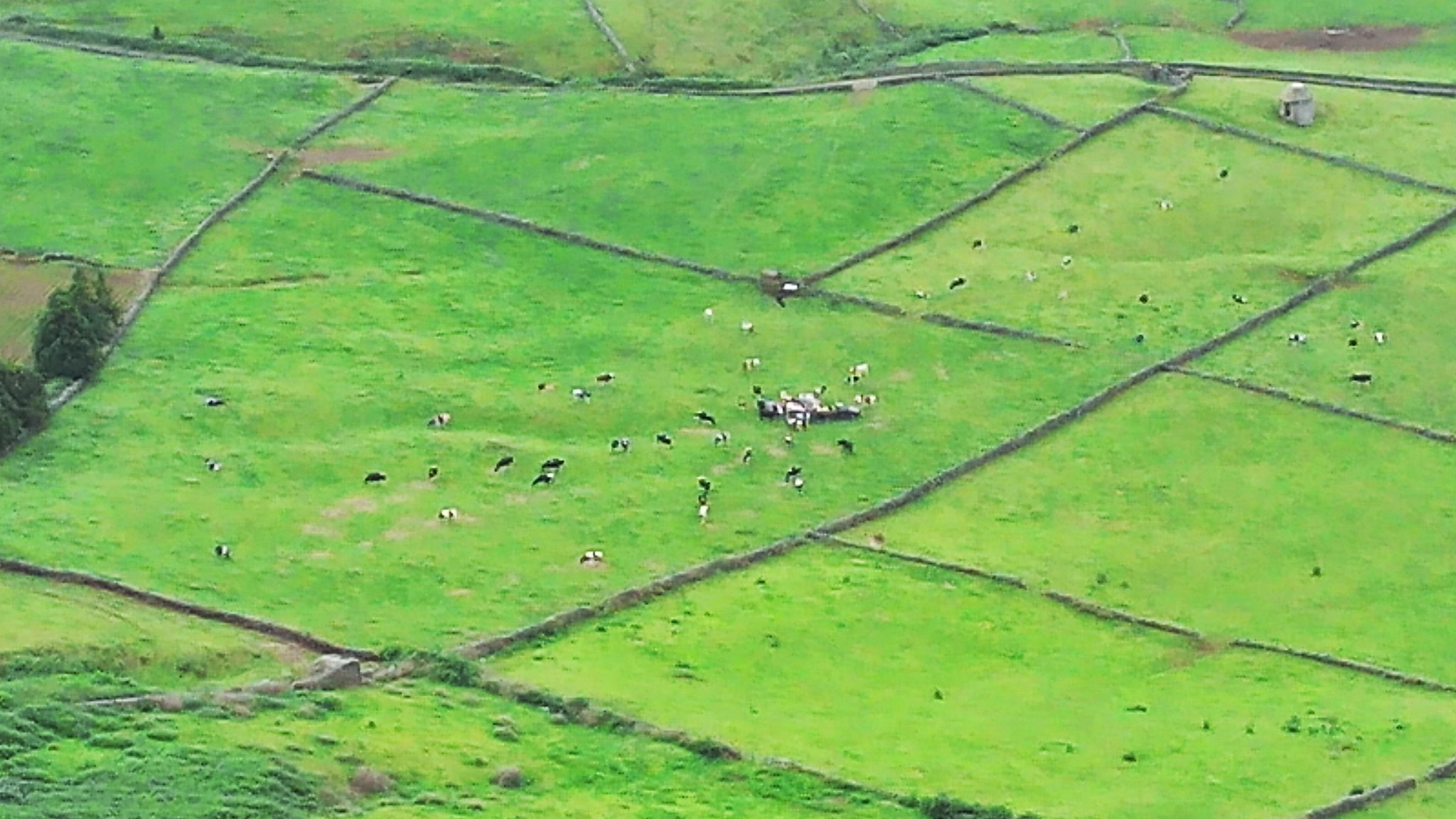This horizontal rectangular image, captured from an aircraft, offers an aerial view of a pastoral landscape below. The green fields are geometrically divided into mostly rectangles and other shapes, likely by fences or stone walls. The largest field, centrally located—cut into a distinctive cone-like shape—is populated with livestock, probably cows, which congregate around a feeder in one corner while others are scattered throughout the grassy expanse. In the bottom right corner, another field hosts fewer animals, distinguishing it from the more densely populated central field. A winding road traces the top boundary of the land, running parallel to the property. Additionally, a small, stone-colored building or cairn-like structure is noticeable in the upper right corner. On the left side of the image, a tilled farm field with a bordering line of trees is partially visible, hinting at the agricultural diversity of the area. Small black and white animals, possibly sheep, are dispersed across some of these fields, grazing peacefully.